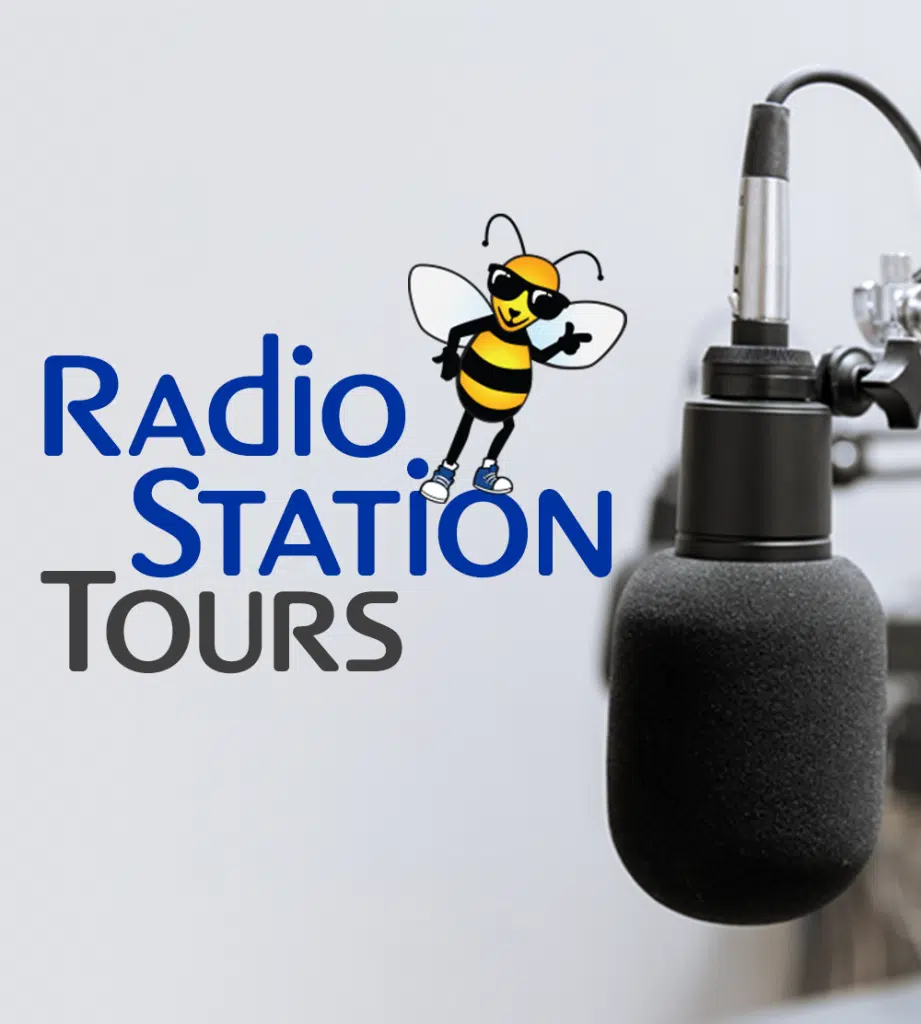The image is a detailed promotional photograph for a radio station named "Tours." The design features a professional studio microphone prominently on the right, with its head pointing downward and a wire attached, indicating it is not wireless. The microphone is positioned to facilitate ease of speaking. The background of the photograph is primarily white, though it may appear slightly blurry. To the left of the microphone, the text "Radio Station" appears in blue lettering, with "Tours" underneath it in black or gray. Adding a whimsical touch, a comic-style yellow and black bumblebee mascot is depicted standing on the letters "I" and "O" in the word "Station." The bumblebee exudes a cool demeanor, wearing dark sunglasses and blue tennis shoes, and is pointing towards the microphone with a finger gun gesture, enhancing the playful and hip vibe of the advertisement.